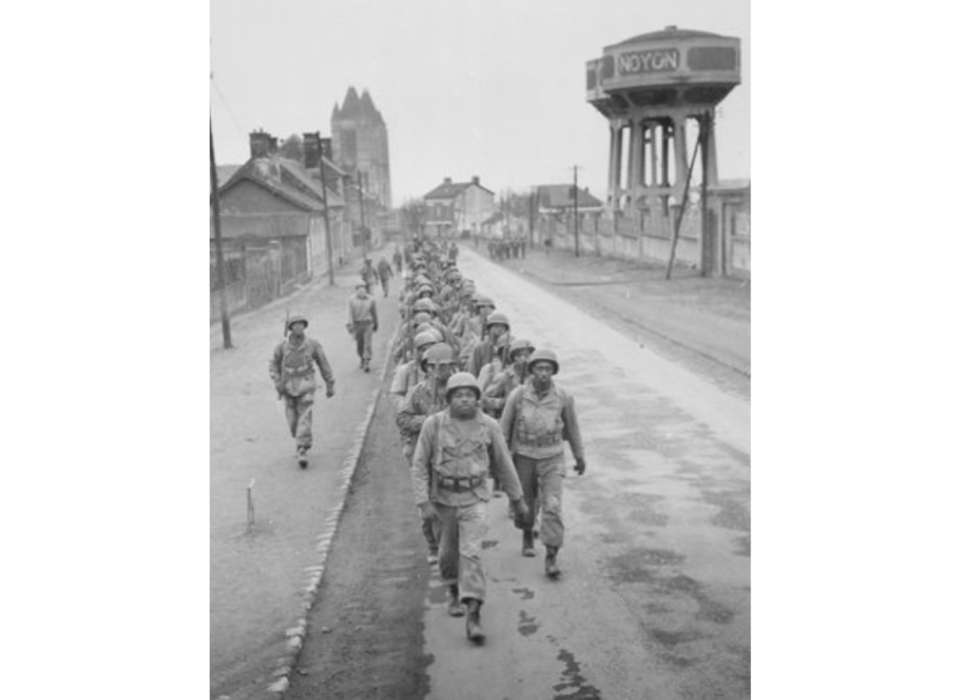In this detailed black and white photograph, we see a column of soldiers marching two abreast along a road, moving towards the viewer. These soldiers are positioned centrally in the image, with an integrated mix of racial backgrounds visible among their ranks. To the left of the marching soldiers, there is a line of officers walking parallel on a sidewalk, and a few scattered soldiers a few rows back. On the right side in the distance, there are two prominent water towers, one of which bears the word "NOYON". The left side of the road features an assortment of older-style buildings, including what appears to be small businesses and a church with a high double steeple. The sky overhead is a muted gray, contributing to the image's somber and historical atmosphere. The scene is evocative of wartime, capturing the soldiers as they march, perhaps towards a battle.